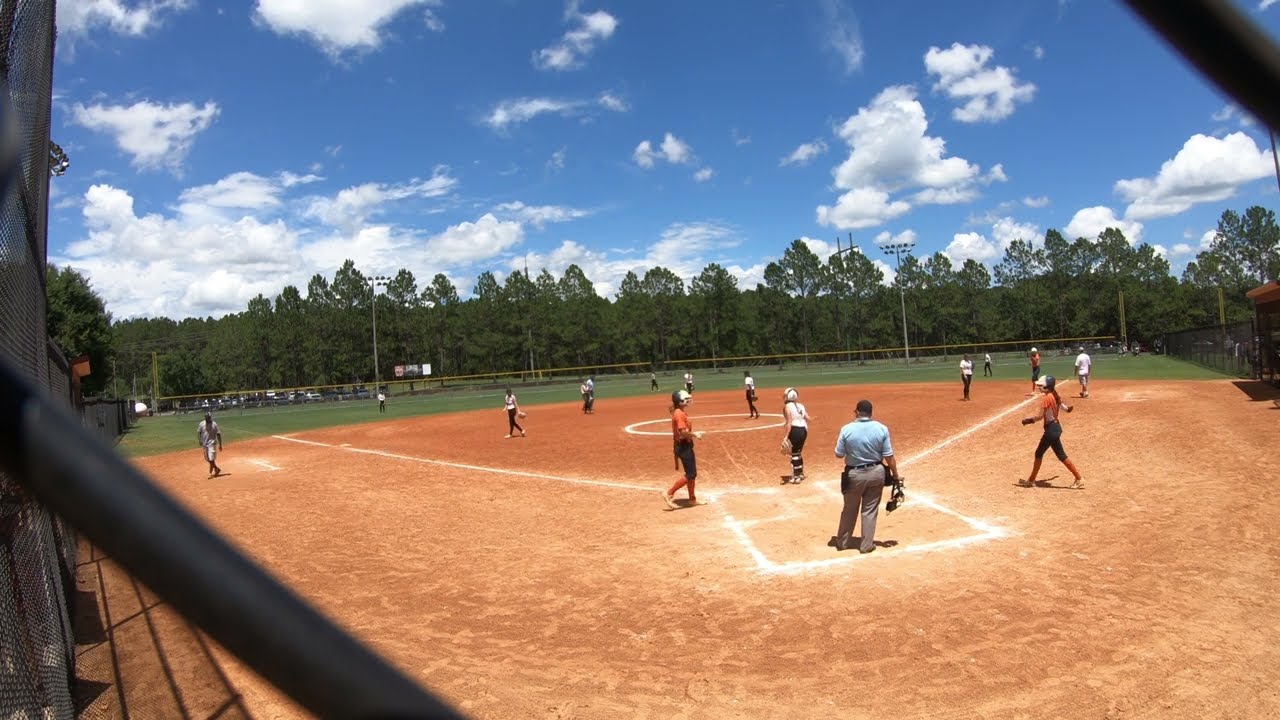The image captures a vibrant and sunny day at a youth women's baseball or softball game, set on a well-defined baseball field with an overhead perspective. The players are dressed in distinct uniforms, with one team sporting orange shirts, black pants, and matching orange shoes, complemented by black and white baseball caps. The opposing team wears white tops, black pants, and white hats. The umpire, clad in official gear, is centrally positioned, holding a facemask, suggesting that the game is in its preparatory stages with players getting into position. The field is marked with white lines illustrating the diamond and bases, while the background features a chain-link fence, a line of trees, and a few cars parked. The sky is a beautiful blue with scattered clouds, enhancing the picturesque, sunny atmosphere of the scene. Sparse with spectators, the image presents a neatly organized, junior amateur league game with a sense of anticipation and community engagement.